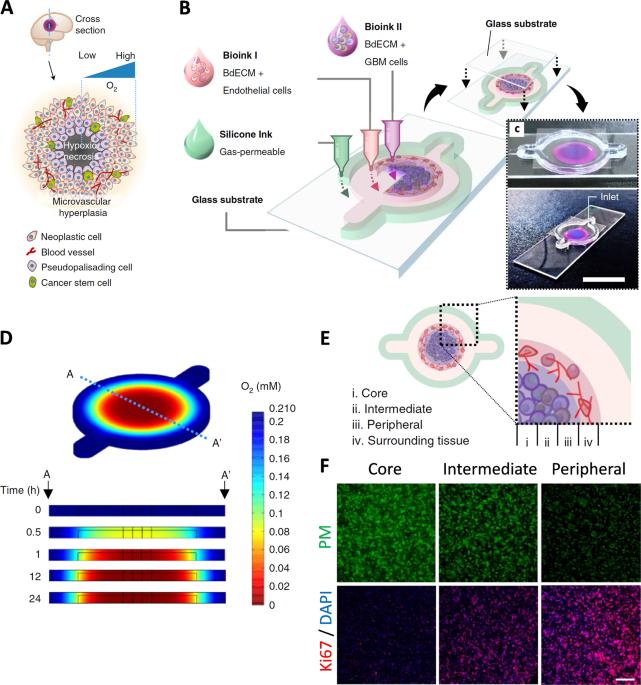The image features a series of biology-related diagrams labeled from A to F, showcasing various cellular and microvascular elements. Starting at the top left, Diagram A displays a cross-sectional view illustrating the presence of neoplastic cells, low-high microvascular hyperplasia, and blood vessels. Adjacent to it, Diagram B includes images that resemble two water drops, labeled with terms like "Bio Inc. 1 BDECM," "Silicon Inc. gas permeable," and "Bio Inc. 2 glass substrate," suggesting the study of cells in various conditions. Moving next, Diagram C shows an image of a glass substrate marked "Intel." 

At the bottom left, Diagram D features a circular diagram in different colors (blue, green, yellow, red) with a color gradient scale ranging from 0 to 0.21, likely indicating heat measurements. In the middle right, Diagram E describes various layers of tissues such as "core," "intermediate," "peripheral," and "surrounding tissue." Finally, at the bottom right, Diagram F depicts a series of six grids, where the matter transitions in color from shades of green in the upper grids to shades of purple in the lower grids, labeled with "core," "intermediate," and "peripheral," likely illustrating stages or zones within a cell culture or petri dish. Additional photos featured include test tubes and microscope plates, providing context to the experimental setup and observations.